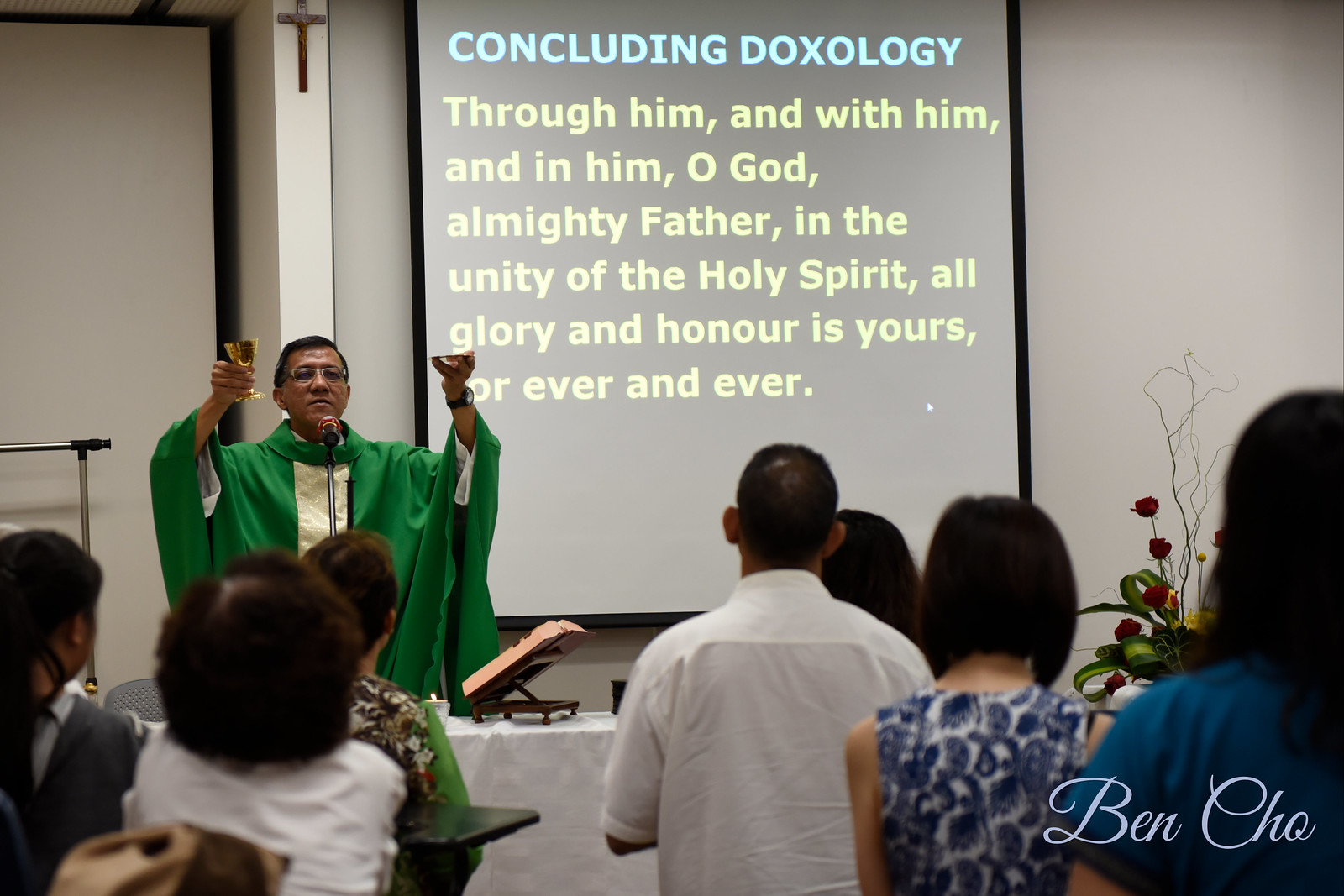The photograph captures a solemn moment during a religious service within a plainly adorned room with white walls. A priest, presumably named Ben Cho, stands front and center in a green robe accented by a white stripe down the middle. He is leading the congregation in the Eucharist, holding a golden chalice in his left hand and a small platter in his right hand. A small cross is affixed high on the wall behind him, and a white screen projects the concluding doxology, which reads: "Through him and with him and in him, O God, Almighty Father, in the unity of the Holy Spirit, all glory and honor is yours forever and ever." In front of the priest, a table is set with a propped open Bible and a lit candle atop a white tablecloth. The audience, a mix of men and women with their backs turned to the camera, stands attentively, engaging in the prayer. Despite the plainness of the room, which could easily be mistaken for an office setting, the reverence of the moment is palpable. A microphone is positioned in front of the priest, suggesting he is addressing a fairly large congregation during this Mass.